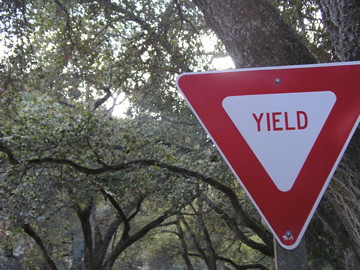This photograph taken outdoors prominently features a red and white yield sign. The sign, constructed from metal and affixed to a gray metal pole, stands at approximately human height. It takes the shape of an upside-down triangle with a red border and a white center, where the word "YIELD" is boldly displayed in red text. The background is filled with large, leafy green trees that stretch across the entire width of the image, giving the impression of a lush, natural setting. The tree immediately behind the yield sign is particularly notable for its thick trunk and vertical reach. While there's some uncertainty, the backdrop may include a body of water, partially obscured by the dense foliage. The sky appears to be overcast, with the sunlight filtered through the canopy of leaves, indicating a potentially cloudy day during either spring or summer.